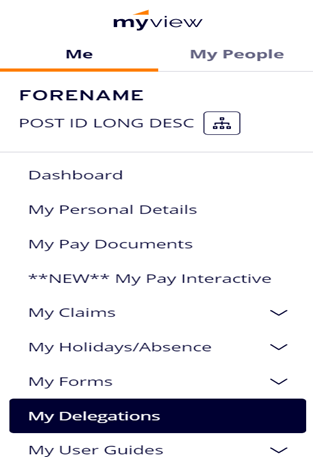The image features a computer interface from the company MyView. At the top, there's an orange triangle pointed to the left. The screen prominently displays the phrase "Me and My People," with "Me" highlighted. Below this title, it lists "foreign name," "post ID long," and "DESC" inside a white box with a grayscale theme.

A gray line runs underneath, leading to a menu with the following options:
- Dashboard
- My Personal Details
- My Paid Documents
- New** (highlighted with asterisks on either side)
- My Pay Interactive
- My Claims (with a dropdown menu)
- My Holidays and Absence (with a dropdown menu)
- My Forms (with a dropdown menu)
- My Delegations (in a black box, no dropdown)
- My User Guides (with a dropdown menu)

The website's background alternates between black for the primary backdrop and white for content areas, creating a predominantly black-and-white color scheme with occasional orange highlights for emphasis.